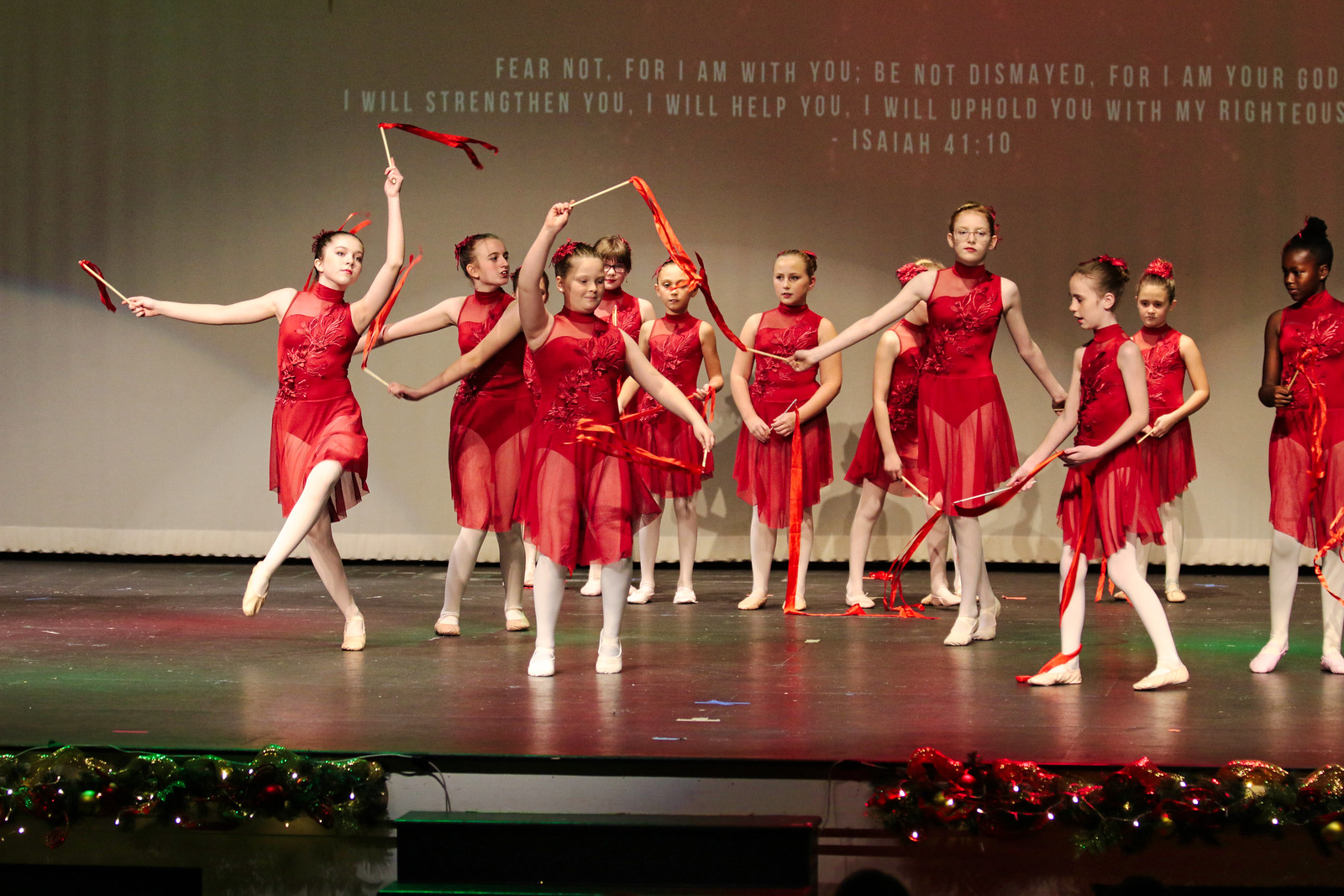The photograph captures a lively scene of a dance recital featuring a group of more than ten young girls performing on a well-lit stage. All the performers are uniformly dressed in red leotard-like dresses with see-through fabric above the chest and on the thigh area, complemented by white stockings and white ballet flats. Each girl holds a stick adorned with red ribbons, adding a dynamic flourish to their coordinated movements.

The stage is intricately decorated, with green wreaths on the left and red-adorned wreaths on the right. Steps leading up to the stage are visible in the lower part of the image. The backdrop features a large white screen displaying a biblical verse from Isaiah 41:10, which reads: “Fear not, for I am with you. Be not dismayed, for I am your God. I will strengthen you, I will help you, I will uphold you with my righteous…” The words fill two lines, with "Isaiah 41:10" cited beneath.

In the forefront, the girl on the far left is particularly animated, extending one stick above her head and the other to her side, displaying a poised and graceful stance. The rightmost girl faces forward slightly angled to the right, her position mirroring the collective harmony of the troupe. Stage lights contribute to the vibrant atmosphere, highlighting the dancers and their carefully choreographed performance.